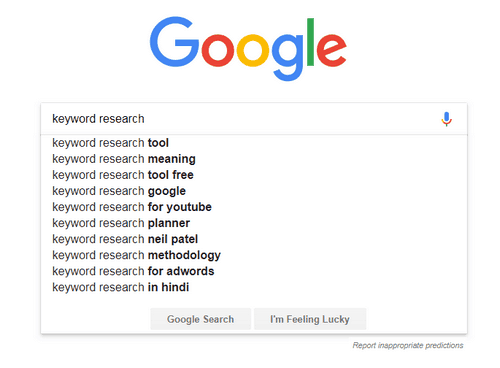The image is a screenshot of the Google search interface. At the top of the screen, the iconic Google logo is displayed with the first 'G' in blue, the first 'O' in red, the second 'O' in yellow, the second 'G' in blue, the 'L' in green, and the 'E' in red. Just below the logo, the search bar shows the query "keyword research" entered, with a microphone icon on the right side of the search bar. Below the search bar, there is a dropdown list of suggested search results starting with "keyword research 2," followed by "keyword research meaning," "keyword research 2.3," "keyword research Google," "keyword research for YouTube," "keyword research planner," "keyword research Leopardo," "keyword research methodology," "keyword research for AdWords," and "keyword research in Hindi." At the bottom of the screen, the typical Google search options "Google Search" and "I'm Feeling Lucky" are visible on the left and right, respectively. Additionally, "Report inappropriate predictions" is found in the bottom right corner.